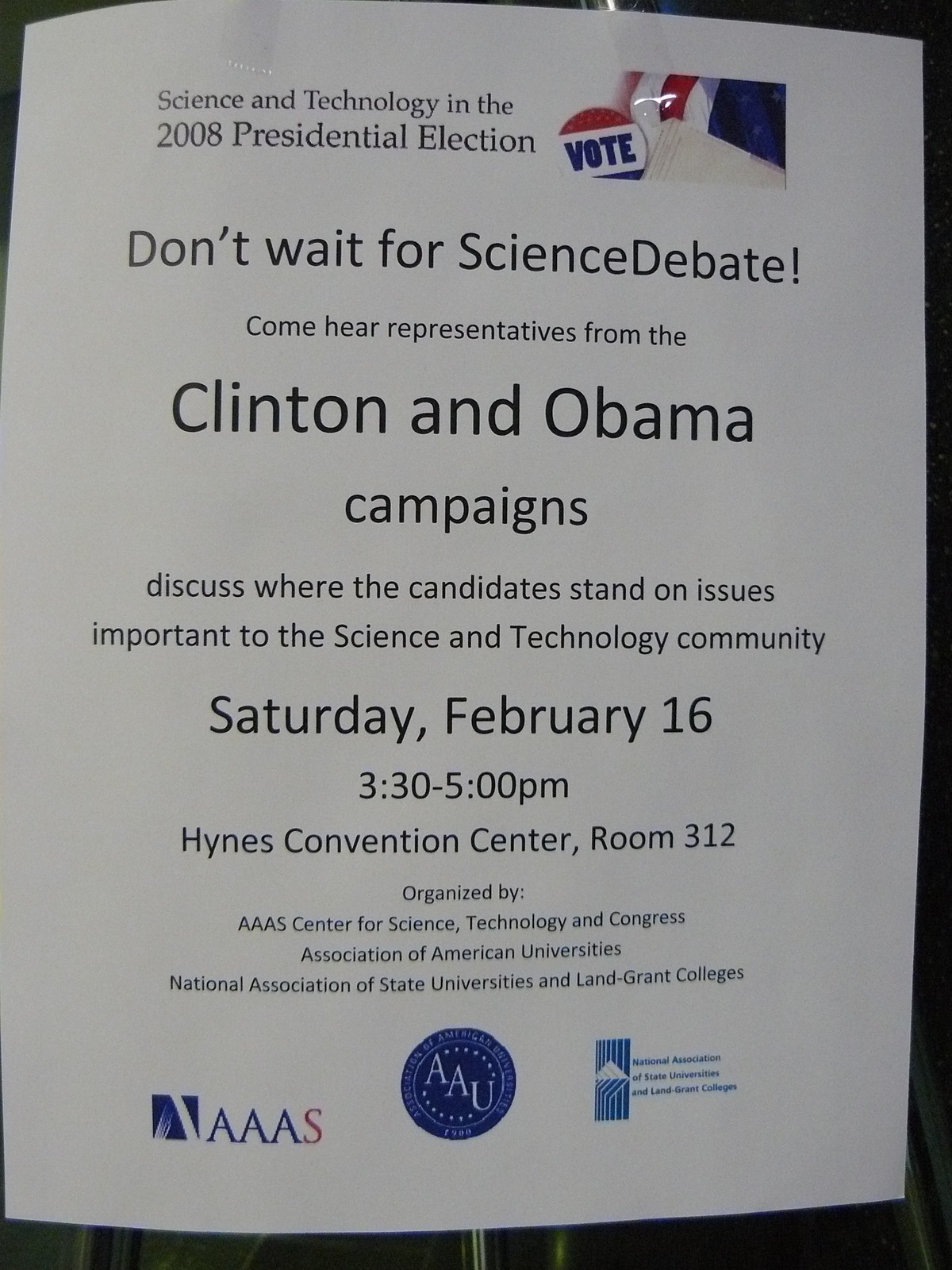This is a tall rectangular photograph of a sign on a piece of paper taped to a wall. The tape is clearly visible at the top, and the wall appears to be a dark green or possibly dark color. The paper has black, red, and blue ink on a white background. At the top left, it reads in bold black letters: "Science and Technology in the 2008 Presidential Election." To the right of this text, there is an image of a portion of the American flag and a vote button colored red, white, and blue that reads "VOTE" in blue letters. Below it, the flyer continues with the text in black letters: "Don't wait for the science debate. Come hear representatives from the Clinton and Obama campaigns discuss where the candidates stand on issues important to the science and technology community." The details of the event are listed as "Saturday, February 16, 3:30 to 5:30 p.m., Heinz Convention Center, Room 312." Additionally, at the bottom of the flyer, there are logos for the AAAS Center for Science, Technology, and Congress, and the Association of American Universities (AAU), along with another unreadable logo.